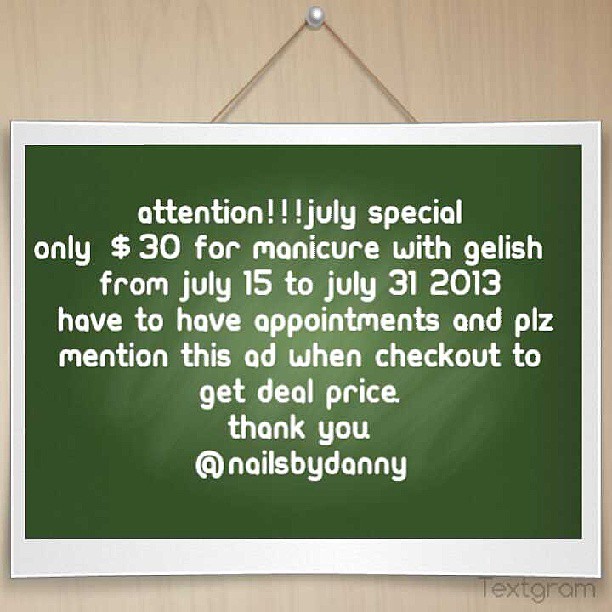This photograph depicts a green chalkboard-style sign with a white border, hanging on a light wooden wall. The sign is suspended by a wire attached to a nail or a thumbtack, which looks like a white pearl. The sign's text, all in lowercase white font, reads:

"attention!!! july special: only $30 for manicure with jellish from july 15th to july 31st, 2013. have to have appointments and plz mention this ad when checkout to get deal price. thank you. #nails by danny."

The details of the light wooden background, the white border, and the precise text create a clear and informative promotional message for a special offer on manicures.